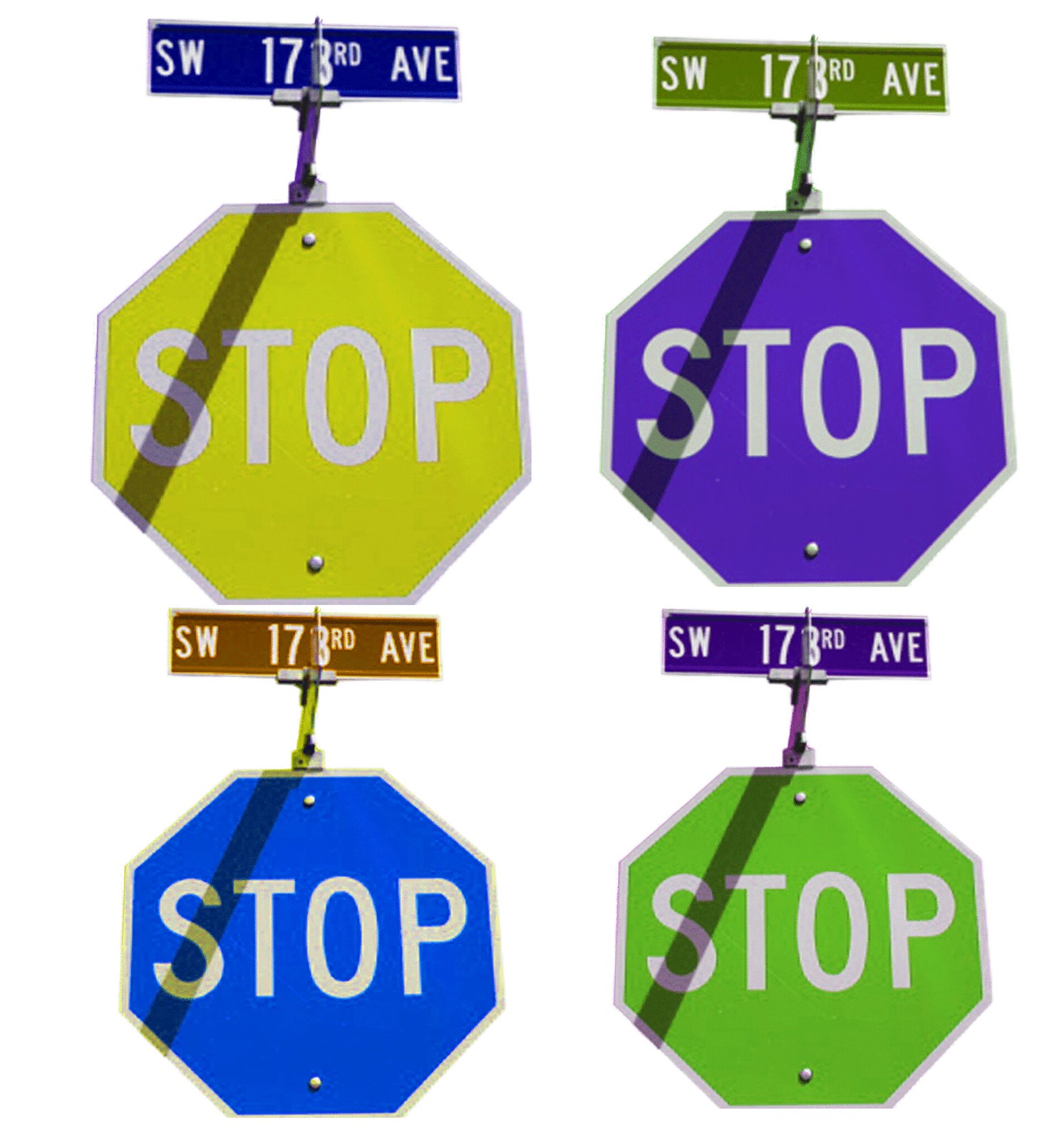This captivating image showcases four uniquely colored stop signs, each paired with a similarly distinctive street name sign. The top left stop sign is a vibrant yellow with the street sign above it in a deep blue, both featuring white text. It bears the inscription "SW 173rd Avenue" with a thin white border. The sign casts a noticeable shadow from its top down to the bottom left angle, intersecting the letters. The adjacent stop sign to the right is a striking dark blue with "SW 173rd Avenue" printed on a green rectangular sign above it. Below these, on the bottom left, is a lighter electric blue stop sign with a matching brown street sign. Finally, the bottom right features a bold lime green stop sign, topped by a dark blue street sign. All stop signs retain their classic octagonal shape with the word "STOP" in stark white letters centrally placed, framed by a white border. Perpendicular street signs are also visible but unreadable due to their angle, adding an element of mystery to this colorful and organized display.